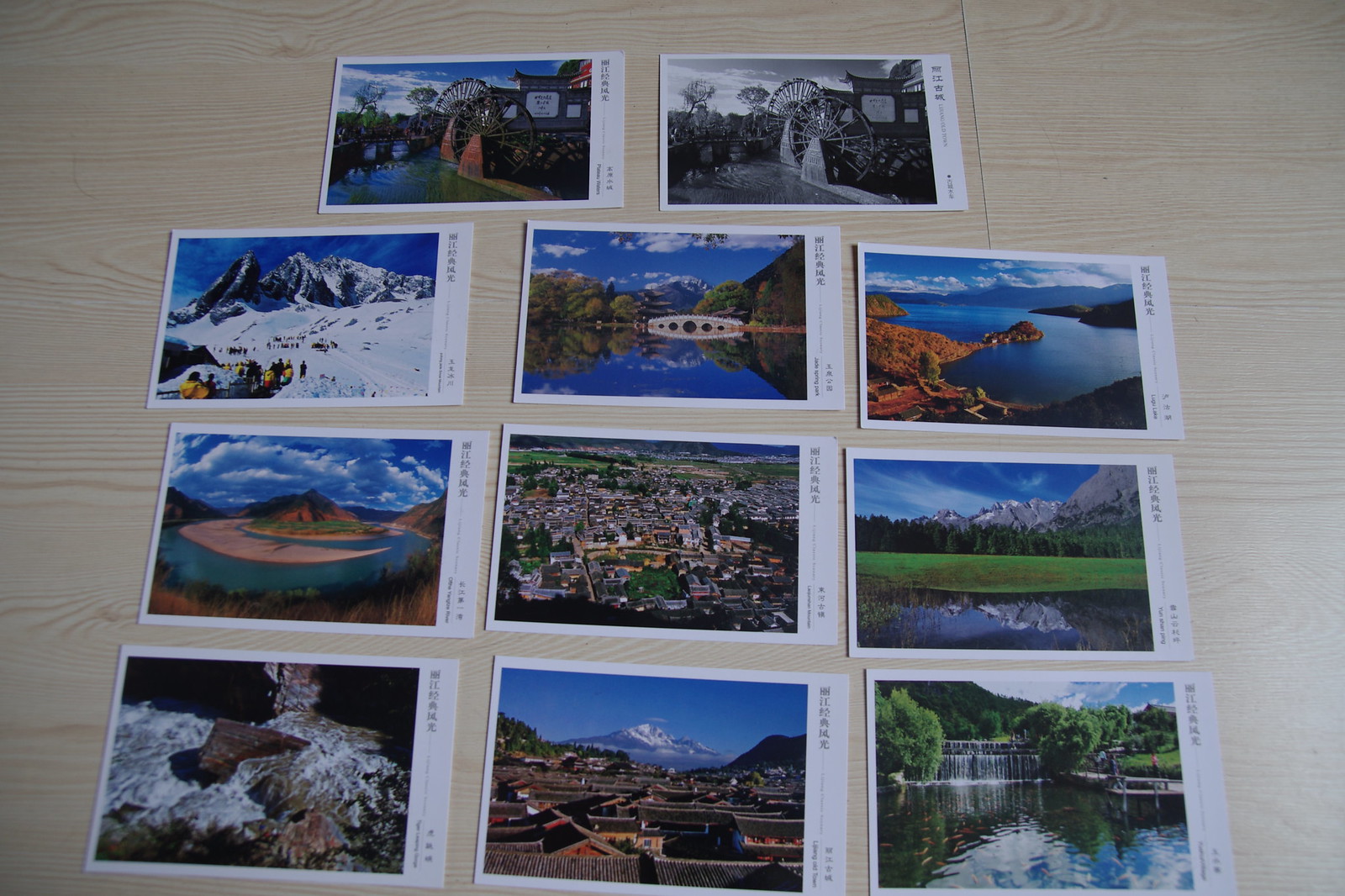The indoor color photograph captures a collection of eleven professionally taken postcards spread out on a light tan, wood-grained surface. The layout forms a grid: the bottom three rows each contain three postcards, while the top row has two centered postcards that stand apart from the rows below. These top two postcards feature the same landscape scene, with one in color and the other in black and white. 

Each postcard showcases a vivid landscape scene dominated by water elements—these include cityscapes with rivers, waterfalls, peninsulas, and large bridges crossing expansive waters. Other prominent features are Ferris wheels, mountain ranges, and bustling cities. Despite the variety of locations around the world, a common visual theme is the presence of water.

The postcards have a distinctive white border on the right side, featuring Asian characters, though no other text or printing is legible. The photograph, while in focus, is poorly lit, allowing the vibrant colors of the landscapes to be the primary points of interest against the pale wooden background.